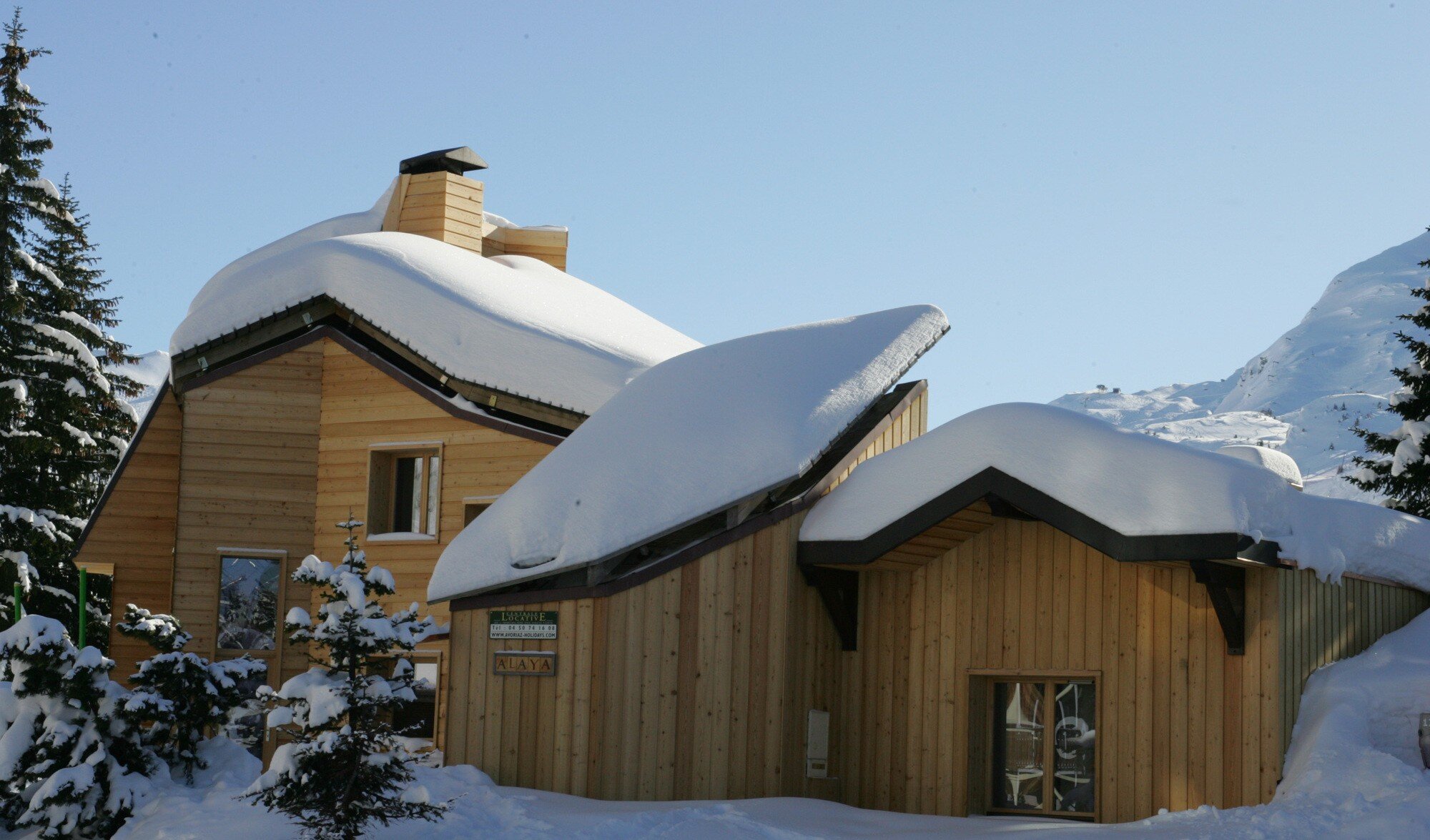The image depicts a high-end modern cabin, possibly situated at a luxurious ski or hunter's lodge, enveloped in a snowy landscape. The sky is clear and light blue, suggesting a bright and crisp winter's day. The structure is composed of multiple sections; two smaller front sections with vertical wooden plank siding and a larger rear section with horizontal siding. The cabin's roofs are heavily blanketed with thick, rounded snow, highlighting the substantial snowfall in the area. Snow covers the ground both in the foreground and background, creating a buried effect.

Flanking the cabin are tall evergreen trees dusted with snow, adding to the wintry ambiance. To the right of the building, a snowy hill rises, while mountains capped with snow loom in the distance. A glass sliding door is situated in the lower right section of the building, and the middle section features two signs mounted on its wall. Various windows punctuate the left side of the cabin, some on the ground floor and others on the second floor, which also includes a chimney on its roof. Overall, the architectural design and choice of materials underline the cabin's high-end and modern aesthetic.